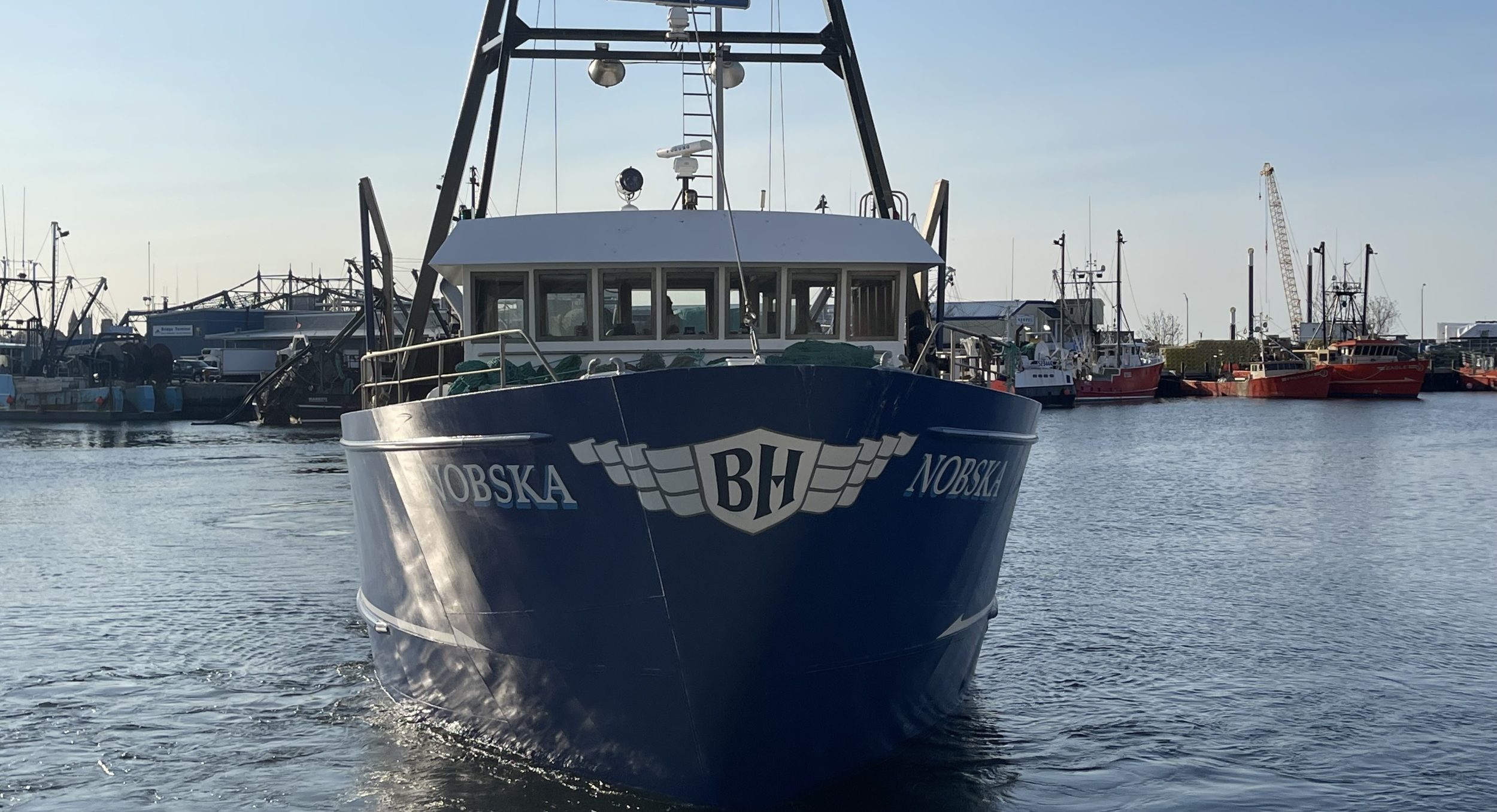This detailed image captures a small blue fishing trawler, named "Nopska," approaching the viewer. The name "Nopska" is displayed on both sides of the boat, and at the very front is a patterned shield bearing the letters "BH" along with decorative banners. The boat features a pilot's house with seven windows and a white roof, and a structure behind the pilot's house equipped with lights and radar. 

The background reveals a busy port area, populated with various commercial vessels, none for leisure or sailing. Among them, a crane is visible on the right side. The sky transitions from a darker blue at the top to a lighter blue and eventually to white near the horizon. The calm body of water, with slight ripples, reflects blue and white hues. The overall scene suggests a regular day at a working dockyard.